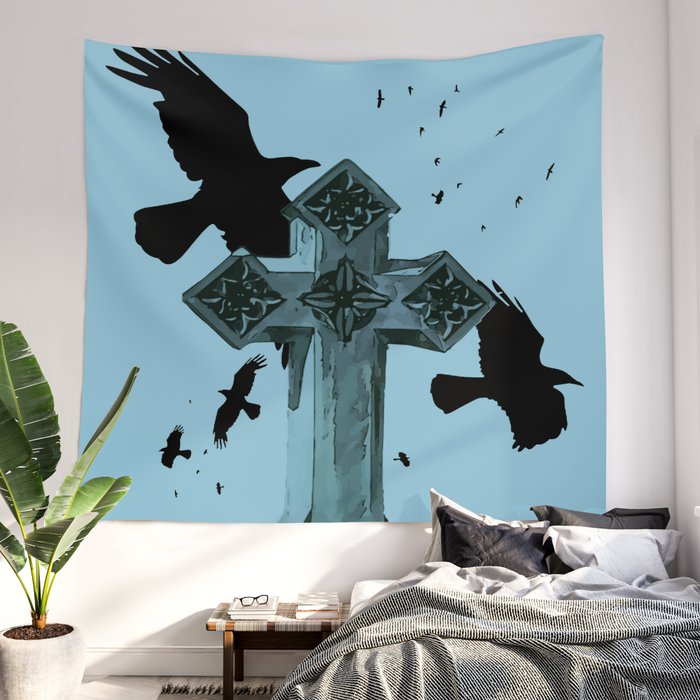The image captures an indoor bedroom scene with soft light grey walls. Dominating the wall is a tapestry with a blue background that features a grey cross at its center, surrounded by numerous black birds that could be eagles, hawks, or ravens. Below the tapestry, on the left side of the room, there is a potted plant with broad green leaves in a white pot. Adjacent to this, a wooden side table with a mixed wood and white top holds a pair of glasses and several books. On the right side of the room is a twin-sized bed, draped with a grey coverlet and white sheets, accented by a set of four pillows in black and white hues. The floor is covered by a tan-grey throw carpet, enhancing the cozy atmosphere of this thoughtfully arranged space.